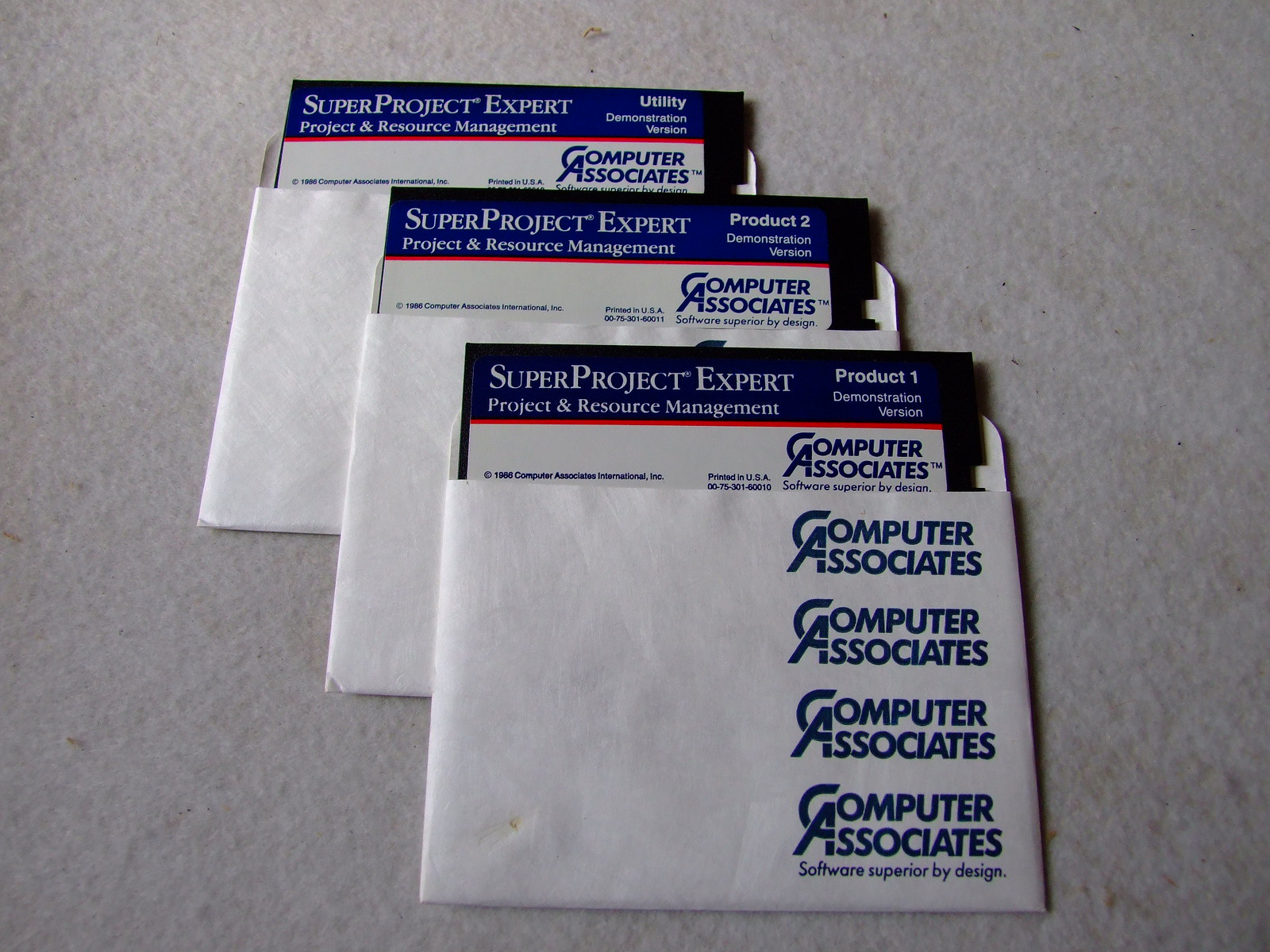This color photograph depicts three vintage floppy disks, neatly placed on a textured white background. Each floppy disk is housed in a white sleeve with "Computer Associates" repeatedly printed in blue along the right side, accompanied by the slogan "Software Superior by Design." The disks partially protrude from their open sleeves, revealing black disks with a red stripe under the logo and labels on a blue background.

The top disk's label reads "Super Project Expert Project and Resource Management," labeled as "Utility, Demonstration Version." The middle disk is marked as "Product 2, Demonstration Version," and the bottom disk as "Product 1, Demonstration Version." Additionally, each disk includes a copyright notice from 1986 by Computer Associates International, printed in the USA with reference number 00-75-301-60010.